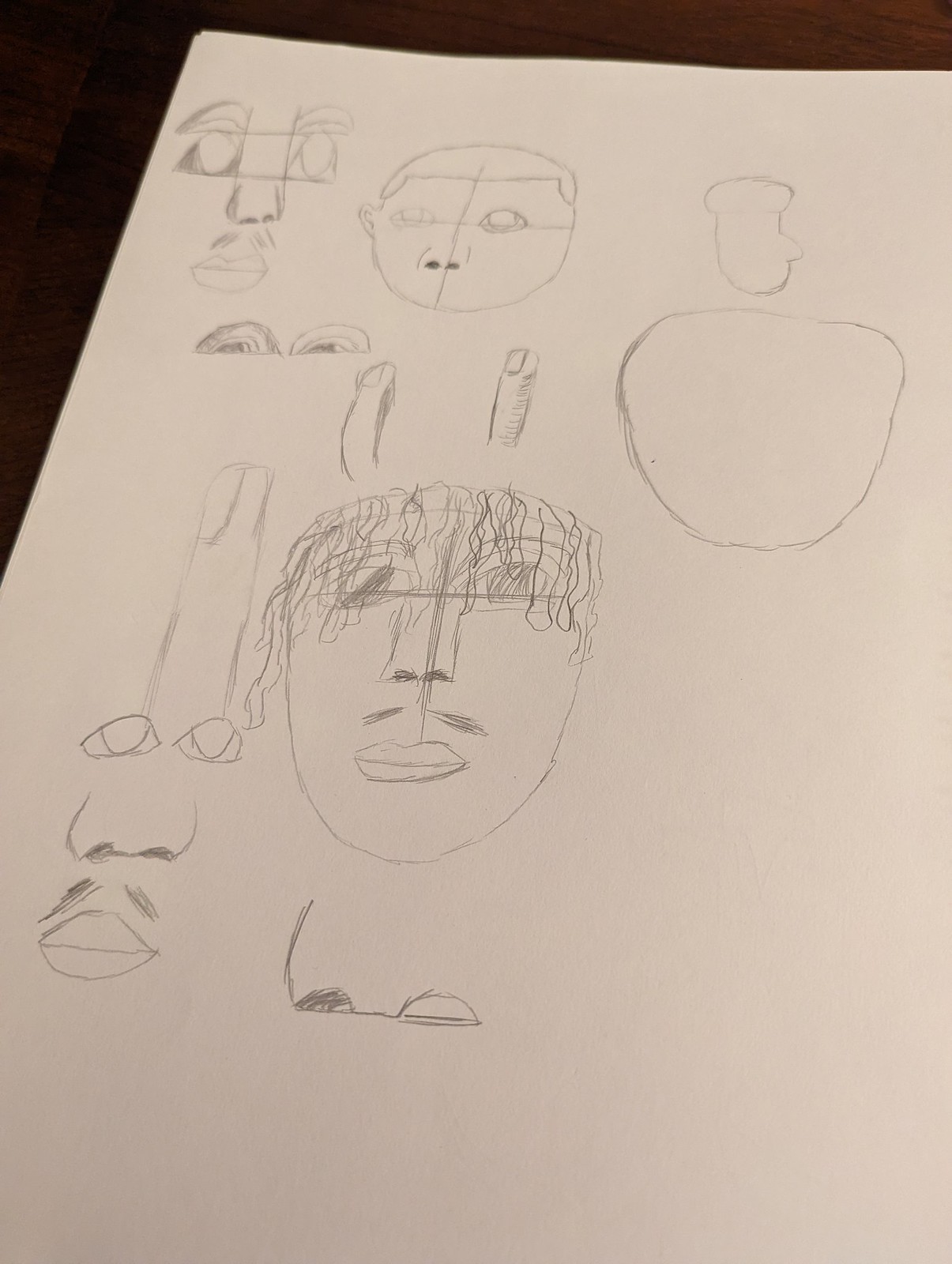The image features a large white piece of paper set against a dark background. The paper displays a detailed pencil sketch that appears to be a work in progress. At the top of the page, the artist is focused on perfecting the facial features, particularly honing the proportions of the nose and eyes. The outline of the face is clearly defined, complete with the shape of the hair and ears. Below, there is an attempt to draw a body which is illustrated in a very round, almost apple-like form. Adjacent to this body sketch, a lightly drawn head shows facial details including hair that drapes over the eyes, a mustache, and lips. Additionally, there is a depiction of a pair of glasses, indicating the artist may be practicing different elements of the face such as the nose, mustache, and lips in multiple iterations.